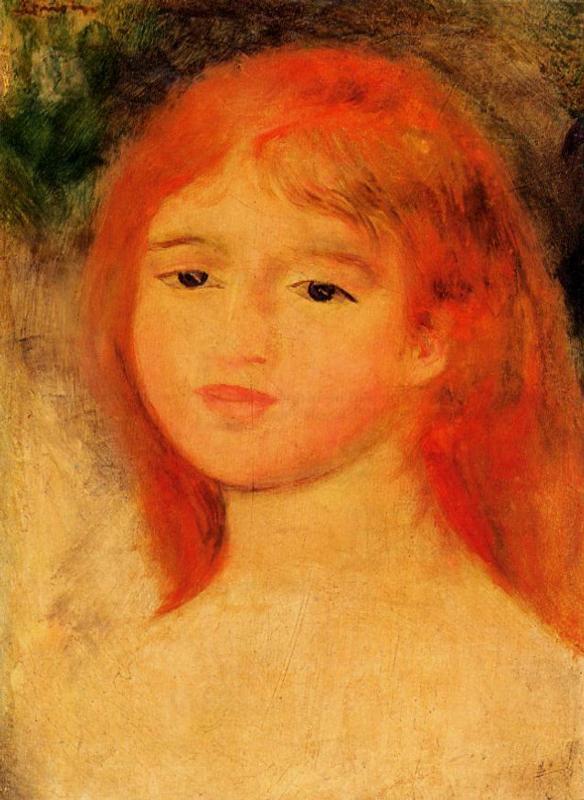A highly detailed light painting captures the face of a young girl with vivid bright red hair that cascades just below her shoulders, partially covering her small ears. She has fair, light yellow-toned skin with a faint blush beneath her ears along her cheeks. Her expression is subtly worried, conveyed through her very dark eyes and slightly downward gaze. Her lips are a distinct pink, adding to her delicate features. The portrait extends from the top of her head to where her neck fades into the background, ending just above her bosom, suggesting she is unclothed. The background features a mix of dark green hues with touches of yellow, brown, and black, accentuating the luminosity of her red hair. A blurred autograph in amber ink is visible in the upper left corner, adding a sense of authenticity and mystery.